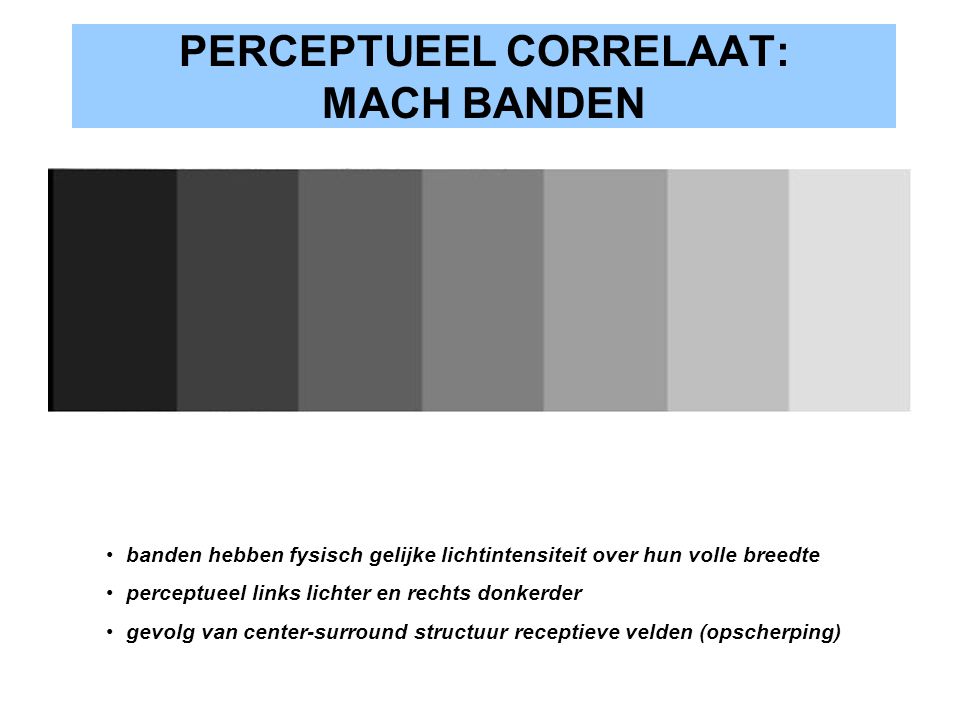The image depicts a rectangular gradient transitioning from black on the left to off-white on the right, segmented into seven different shades of grey. At the top of the image is a light blue rectangle containing German text, which appears to serve as a label or title, reading "Perceptual Correlate Match Abandon." Below this title, the segmented gradient features distinct bands of grey, ranging sequentially from dark grey to medium grey to lighter grey shades. Underneath the gradient are three bullet points, each with additional German text, with the first mentioning terms such as "Banden, Heben, Fiesch, Jellig, Lichtenstein, Overhahn, Wohlbritt," the second listing "Perceptual, Links, Litscher, Rex, Dankter," and the third including "Jevolg van Center, Surround, Structure, Receptive, Lewelden," followed by "Abscherping" in parentheses. This gradient scale seems to serve a purpose related to adjusting or calibrating visual brightness, potentially for a television or other display device. The background of the image is white, which contrasts with the elements to enhance clarity.